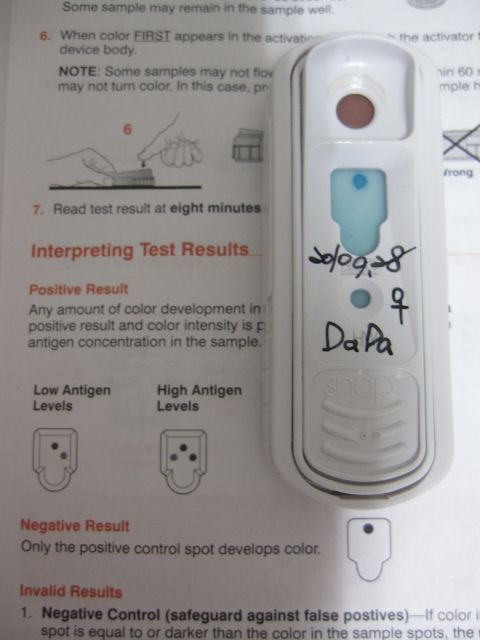The image depicts detailed paperwork related to antigen testing, featuring a specific section on interpreting test results. Prominently centered on the paper is an oblong plastic device used for antigen testing. The device has an indented red circle at the top and a blue square beneath it, which terminates in a circle. Within the blue square, near its top, there is a notable blue dot. This testing device is marked with a female symbol, characterized by a circle intersected by both a vertical and horizontal line, and also bears the text "DAPA."

Accompanying the testing device, the paperwork, predominantly white with red headings and black text, elaborates on the interpretation of antigen test results, distinguishing between low-level and high-level antigen indicators. The document details that invalid or negative results occur when the color spot contrasts significantly in shade, with examples provided showing a light blue tone compared to a dark blue tone. This comprehensive documentation aims to assist in the accurate analysis of test outcomes, ensuring clarity between different antigen levels and possible result discrepancies.